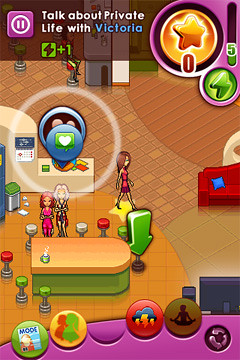The screenshot depicts a scene from a mobile game, focusing on a young female character with long brown hair, dressed in a red dress. A yellow star beneath her feet indicates that she is the player's character. A green arrow points towards the next objective. The setting is a cozy cafe-bar area featuring a green-based table with a wooden top, surrounded by bar stools in red, white, and green colors. Two other female characters are present in the scene. A small trash can is visible in the corner, contributing to the detailed environment.

At the bottom of the screen, there are several icons representing different in-game features: a magazine, two silhouettes, stormy clouds, and a yoga pose. In the upper right corner, the game displays stars with the count at zero and a lightning bolt with five units. A prompt instructs the player to "talk about private life with Victoria" for one lightning bolt.